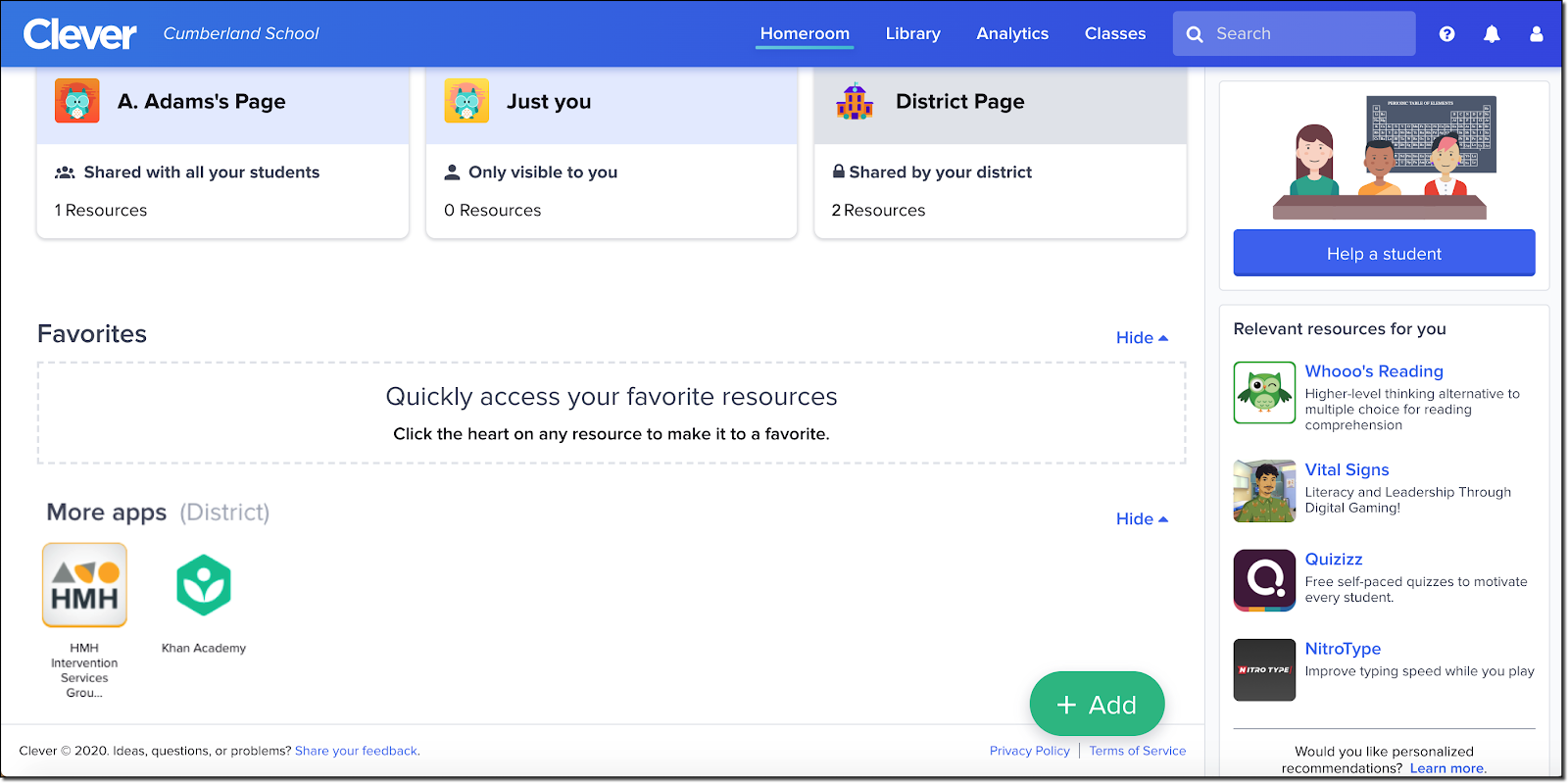The image depicts a webpage with a structured layout. At the top of the page is a prominent blue bar featuring the word "Clever" in bold, white text. Below this, a light blue bar spans about a quarter of the page, labeled "Adam's Page". Adjacent to this label is a small thumbnail image. This light blue bar is followed by another similar bar titled "Just You", also with a thumbnail beside it. The next section is "District Page", presented on a light gray bar, again accompanied by a thumbnail.

Under each heading, there's brief information about the sections. "Adam's Page" indicates it is shared with all students and includes one resource. "Just You" is only visible to the user with zero resources. "District Page" is shared by the district and contains two resources.

The bottom quarter of the page features a graphic of three students—a white girl, an African-American boy, and an Asian-American boy—seated together at a desk. Below this image is a blue bar with the text "Help a Student" in white. Following this bar, there is a section titled "Relevant Resources for You" listing resources such as "Who's Reading," "Vital Signs," "Quiz," and "Nitro Type."